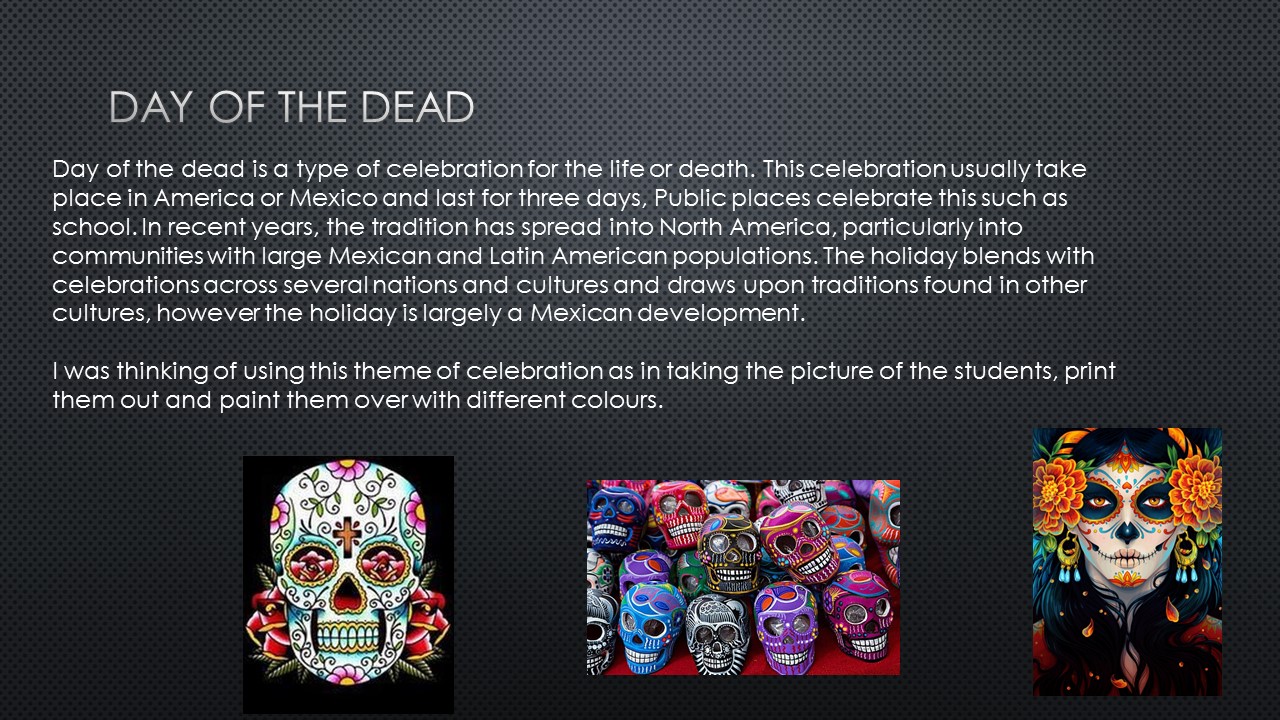This detailed PowerPoint slide themed around the Day of the Dead features a textured black and gray background, prominently overlaid with descriptive text about the holiday. The central text outlines the cultural significance and widespread celebration of the Day of the Dead (Día de los Muertos), highlighting its origins in Mexico and its spread into North American communities, particularly where there are large Mexican and Latin American populations. The text explains that this celebration of life and death typically lasts for three days and is observed in public spaces like schools.

At the bottom of the slide, three vibrant, colorful images depict various aspects of Day of the Dead artistry. On the bottom left, there is an elaborate illustration of a sugar skull adorned with intricate designs in whites, reds, pinks, yellows, greens, purples, blacks, and oranges. The skull features an upside-down heart for a nose and is decorated with pink flowers and leaves. 

The center image displays a collection of decorated wooden skulls stacked closely together. These skulls are painted in a multitude of colors, including purple, blue, black, pink, and dark blue, capturing the festive and eclectic spirit of the celebration.

On the bottom right, there's a striking digital illustration of a woman wearing Day of the Dead makeup. Her face is painted to resemble a sugar skull, with details such as dark eyes, a nose resembling a cat’s, and whisker-like decorations. Flowers adorn both sides of her face near the eyes, and she appears to be wearing headphones.

The overall theme of the slide emphasizes the celebration through art and suggests an interactive project idea: taking photos of students, printing them, and painting over them with an array of vibrant colors to embody the festive spirit of the Day of the Dead.